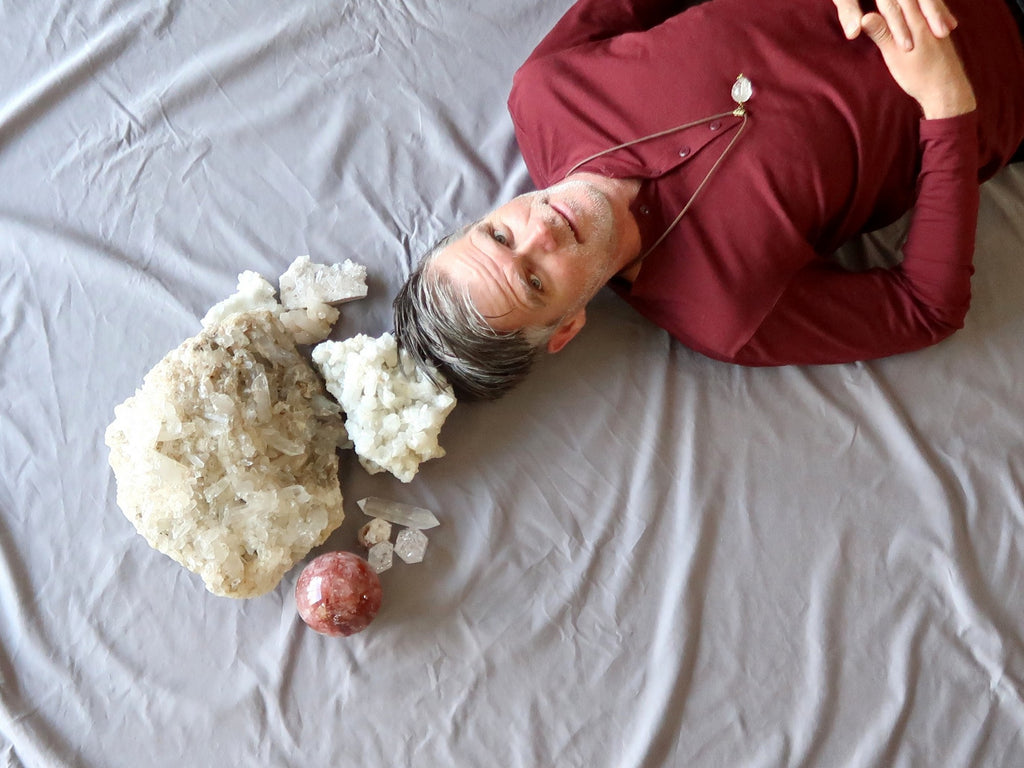A man with slicked-back grey hair and light eyes is lying diagonally on a bed with a light grey, wrinkled sheet. He is wearing a red, long-sleeved polo shirt with half buttons and a golden necklace that features a small pendant resembling a watch or possibly a crystal. The man, whose hands are clasped on his stomach, is looking up thoughtfully with a slight smile on his face. Arranged around his head are various minerals and crystals: directly behind his head is a medium-sized white rock, accompanied by several quartz pieces, including an oblong one and a large quartz cluster. Close to these is a polished red spherical stone. There are also beige and additional white crystal-like rocks nearby, suggesting a New Age or ritualistic setting.